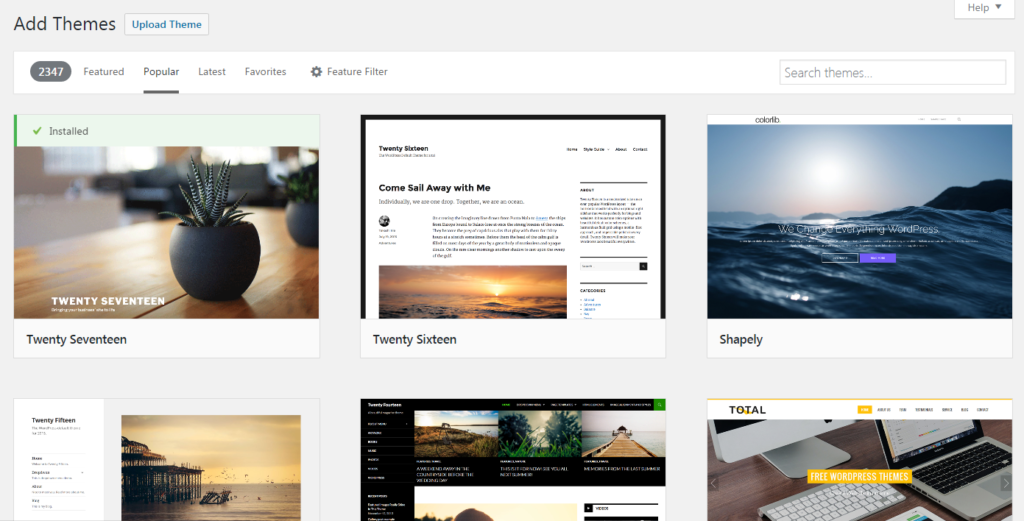The image showcases a screenshot of a website builder platform, akin to WordPress or Wix, which enables users to create and customize their personal websites without requiring any web development skills. The interface has a clean, light gray and white background.

In the top left corner, bold black text reads "Add Themes," and next to it, in smaller blue text, is the option to "Upload Theme." Centrally located on the page are several sample images, each accompanied by descriptions that showcase different website themes, such as "2017," "2016," and "Shapely." These images provide a visual preview of how a website might appear when using these themes. Clicking on any of these theme samples redirects the user to a detailed page with more images, information, and potentially the option to purchase the theme.

At the top center of the interface, navigation links direct users to various sections of the website. The left-hand side features a gray circle with white text displaying the numbers 2, 3, 4, and 7. Adjacent to this, in gray text, are category links labeled "Featured," "Popular," "Latest," "Favorites," and "Feature Filter." The "Popular" category is underlined with a gray line, indicating it is the currently active page being viewed.

In the top right corner, there is a search bar with placeholder text, "Search Themes," allowing users to search for specific website themes.